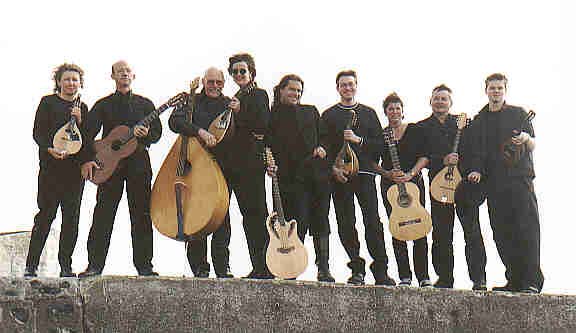In this outdoor photograph, nine musicians are standing on a concrete ledge under a bright white sky, suggesting sunlight overhead. The group consists of six men and three women, all dressed uniformly in black clothing, including black pants, long-sleeve shirts, jackets, and some wearing sunglasses. Each musician is holding an acoustic instrument—there are a couple of guitars, about three mandolins, and other large stringed instruments that resemble a cello or bass. They are arranged in a linear row, facing the camera and smiling. Notably, the gentleman in the middle stands out with his long dark hair and tall black boots.